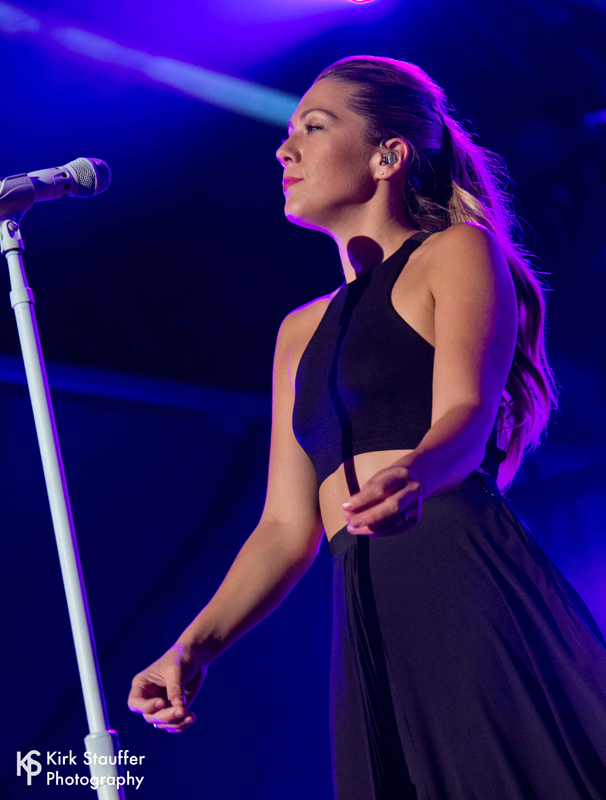This detailed image depicts a young white female singer, standing on stage in an indoor setting. To her left is a black, standard microphone mounted on a whitish-gray mic stand. The singer, with her long, blonde hair styled in a ponytail that reaches her waist, is facing the audience to her left. She is wearing a black halter-neck top that exposes her midriff and has a long, black skirt or gown on her lower torso, though the length is cut off in the frame. Her arms are extended out, making gestures as if snapping, adding an expressive flair to her performance. She has a serious look on her face, with red lipstick adding a pop of color. An earpiece is visible in her ear, along with barely visible earrings. The stage background is dark, illuminated by a pinkish glow from above. In the bottom left corner of the photo, a watermark reads "Kirk Stouffer Photography."